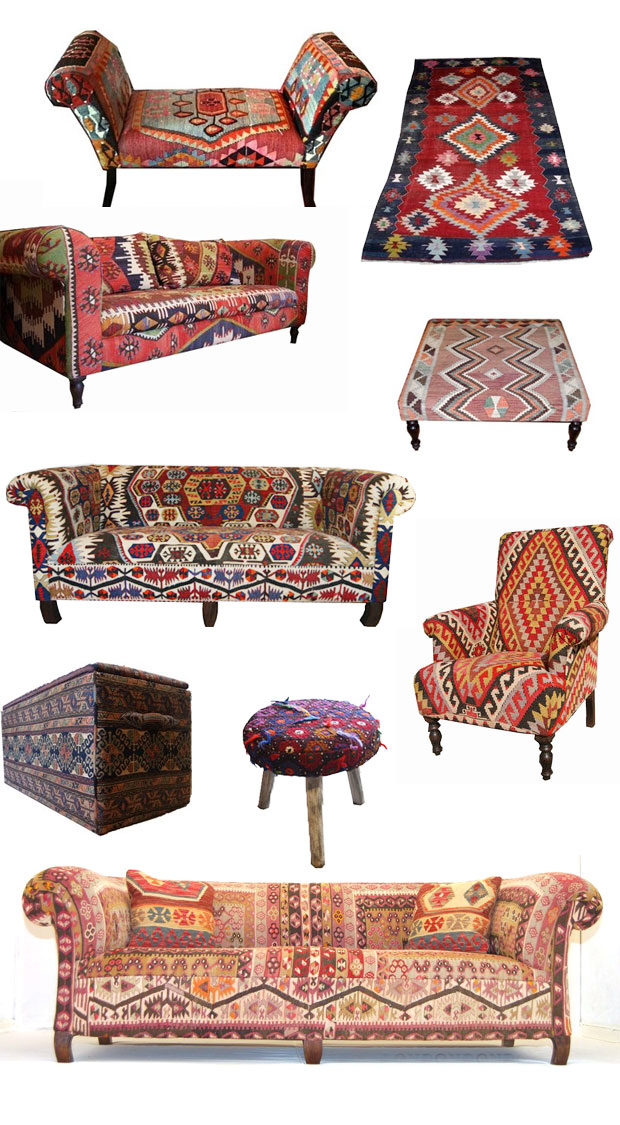The photograph showcases an eclectic and vibrant assortment of furniture and decor, blending modern and traditional elements. Dominating the scene are several brightly colored sofas, armchairs, and loveseats adorned with an array of decorations and intricate patterns. One armchair features Native American-inspired designs in red, brown, and yellow, while another sofa sports a palette of black, red, and white with three decorative cushions. The vivid red sofa stands out with its striking designs.

A long, multicolored rug runs across the floor, framed by a dark blue border. Inside, a red rectangle houses multifaceted diamond shapes with layers of beige, blue, orange, pink, and red. This intricate pattern is mirrored on a large predominantly red loveseat and a smaller beige loveseat.

The room also includes a variety of stools and benches, each uniquely styled. One footstool showcases red flowers on a knitted cushion, while another features a zigzag pattern of cyan, white, brown, green, and pink. A third, resembling a pincushion, combines purple, pink, red, and orange on three wooden legs.

Adding to the ensemble is a long wicker chest, described as brown and complementing the colorful array of fabrics. The overall effect is a harmonious blend of colorful, richly decorated textiles in a space filled with character and cultural motifs.